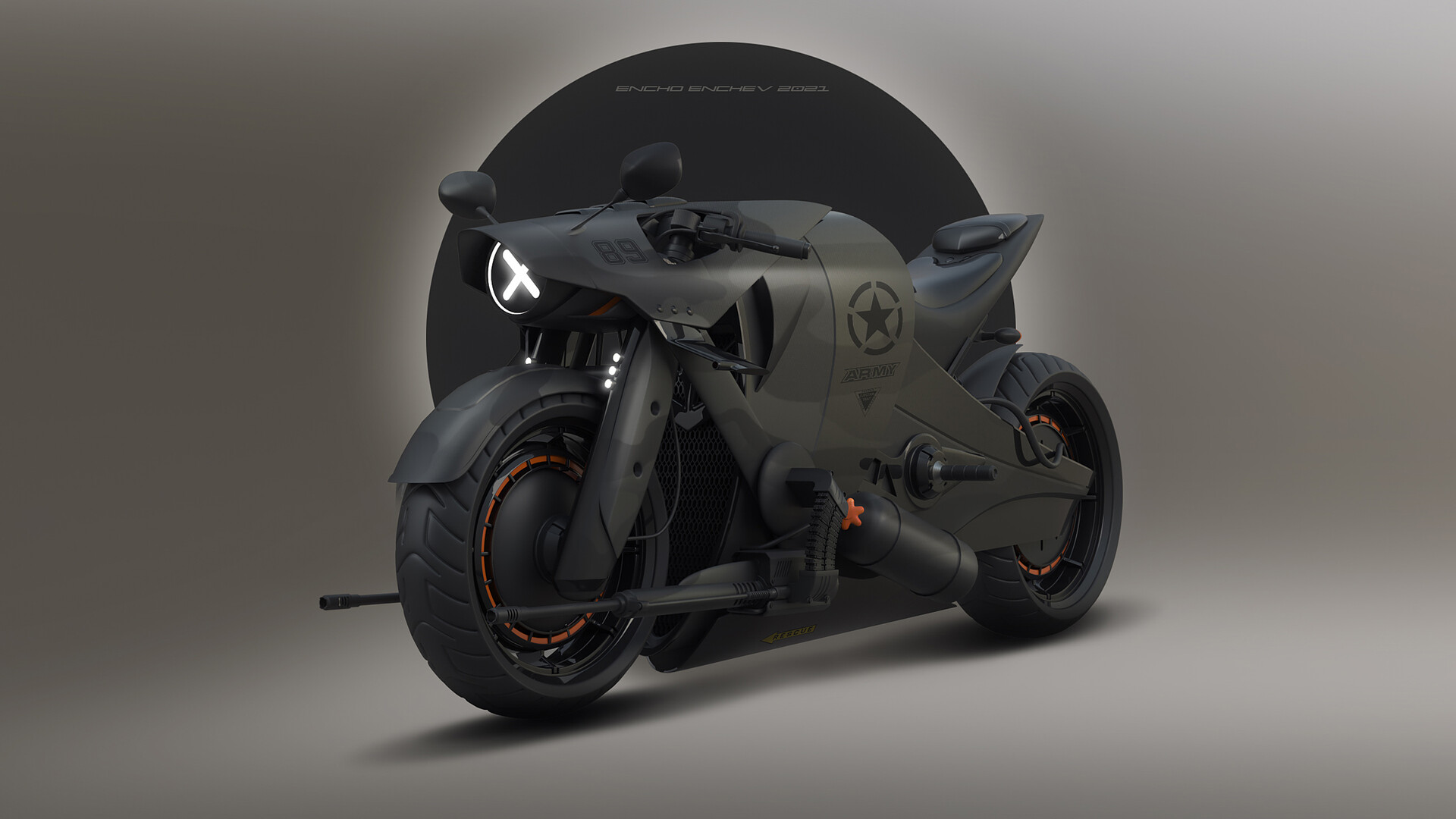The image is a striking advertisement for a futuristic motorcycle, rendered in 3D with a sleek and modern design. The motorcycle, which occupies the central focus of a rectangular frame, has an aggressive, sports-type appearance with sharp lines and a matte black finish accented by slim orange details around the rims and a noticeable orange gas cap lid. This high-tech bike also features camouflaged grey and green patterns, giving it a stealthy aesthetic.

Positioned on a grey surface with a dark grey circular backdrop, the motorcycle commands attention with its large black wheels and distinctive black and orange rim accents. Notably, dual gun barrels are mounted on either side near the footrests, enhancing its intense, almost combat-ready look. The headlight is uniquely illuminated with an 'X' symbol, and a prominent black star within a segmented circle is displayed on the side of the motorcycle. Above the bike, the text "Enchev 2021" is clearly visible, further branding this concept art piece.